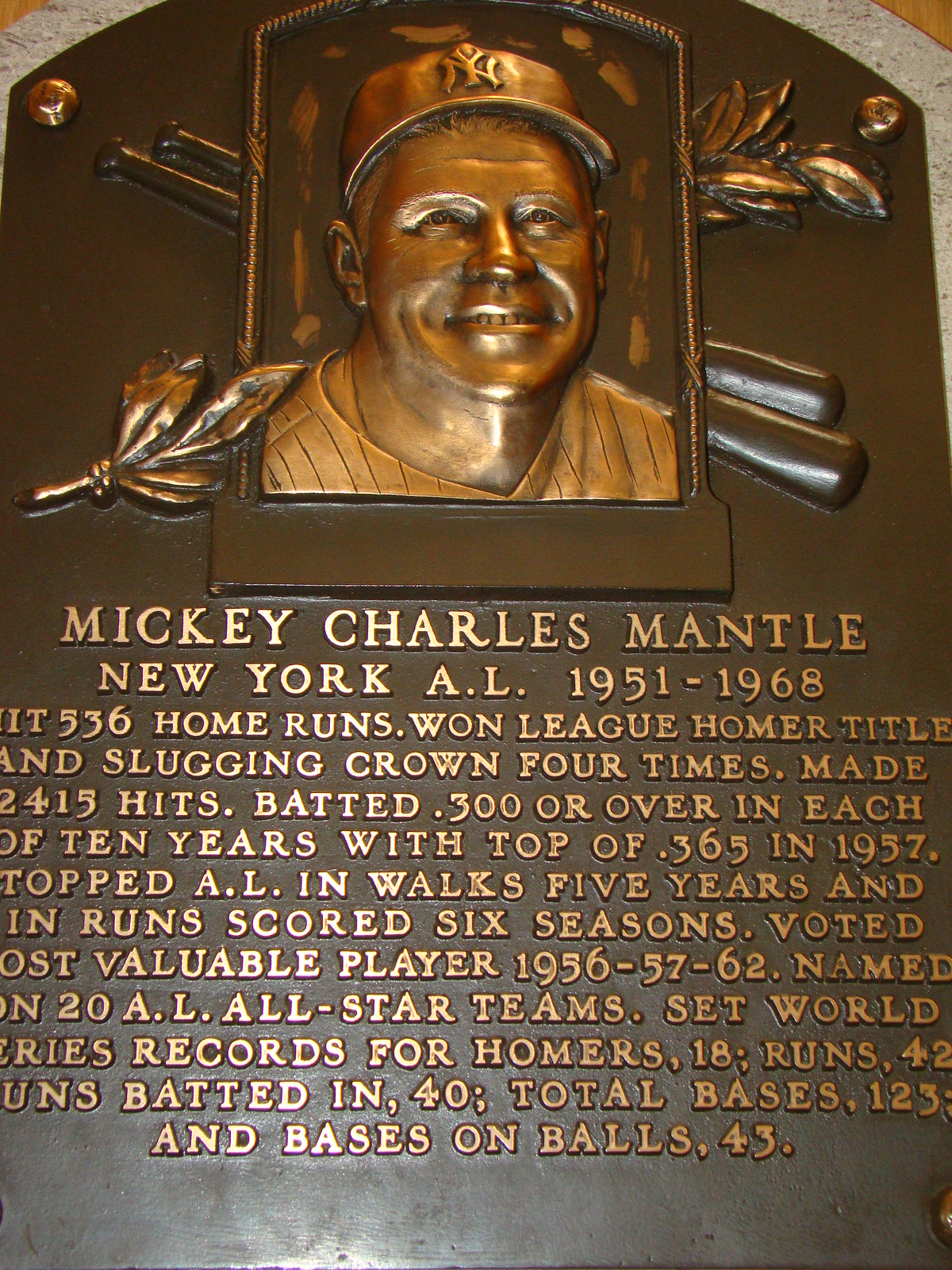This detailed bronze plaque honors the celebrated baseball player Mickey Mantle. It features a polished, embossed silhouette of Mantle donning his iconic Yankees hat, smiling, and encircled by decorative elements including two baseball bats and leaves. The plaque notably resides in the Hall of Fame or at Yankee Stadium, marking Mantle's legendary career with the New York Yankees from 1951 to 1968. In golden text below his likeness, the plaque chronicles his monumental achievements: 536 home runs, a league homer title, and four slugging crowns. It highlights his impressive 2,415 hits, a consistent batting average of .300 or higher over ten years with a peak of .365 in 1957. Mantle led the league in walks five times and in runs scored six times, earning the title of Most Valuable Player in 1956, 1957, and 1962. He was named to 20 All-Star teams and set World Series records for 18 home runs, 42 runs, and 40 runs batted in. The inscription, although partially cut off, emphasizes Mantle's enduring legacy as one of baseball's greatest players.